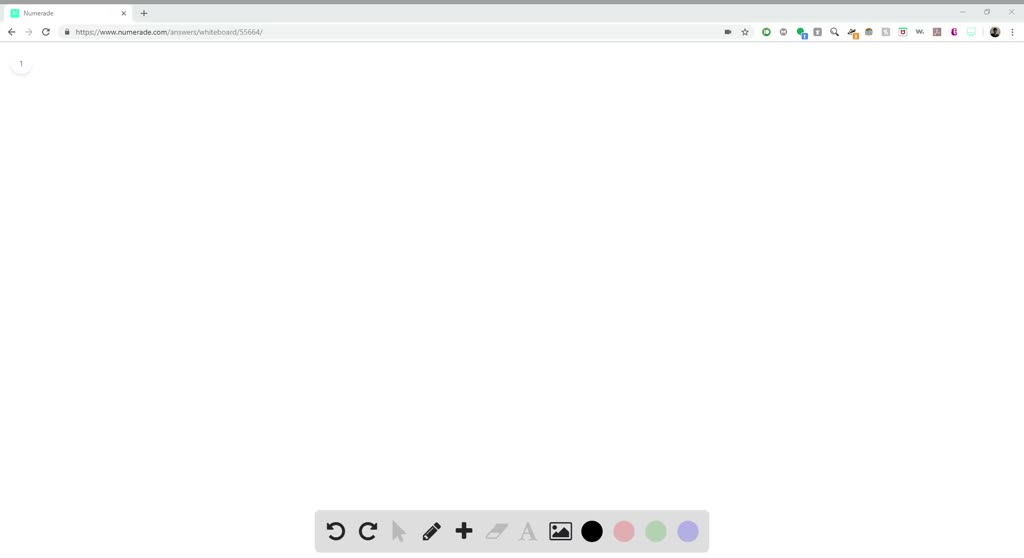The image depicts a mostly empty website displayed as one tab in a web browser. The tab reads "Numerade" in gray text on a white background, accompanied by a green square to the left. On the right side of the tab is an "X" icon to close it. Below the tab are standard browser navigation buttons, including left and right arrows, a refresh icon, and the URL "https://www.numerade.com/Answers/Whiteboard/55664/."

To the right of the URL bar, there is a collection of icons: a star, a green circle, a gray circle, a Facebook icon with a green circle, a nondescript gray square, a magnifying glass, a yellow square containing the number '1,' an unidentified icon, a gray square with white detailing, a browser icon, an icon displaying 'W,' an Adobe PDF icon, a purple icon, a green icon that is unclear, and a circular profile picture icon, albeit too small to discern clear details.

Below the web address, the main part of the screenshot shows a large, blank whiteboard space that appears to offer various drawing tools. Additional navigation buttons include another refresh button, and "Go back" and "Go forward" options.